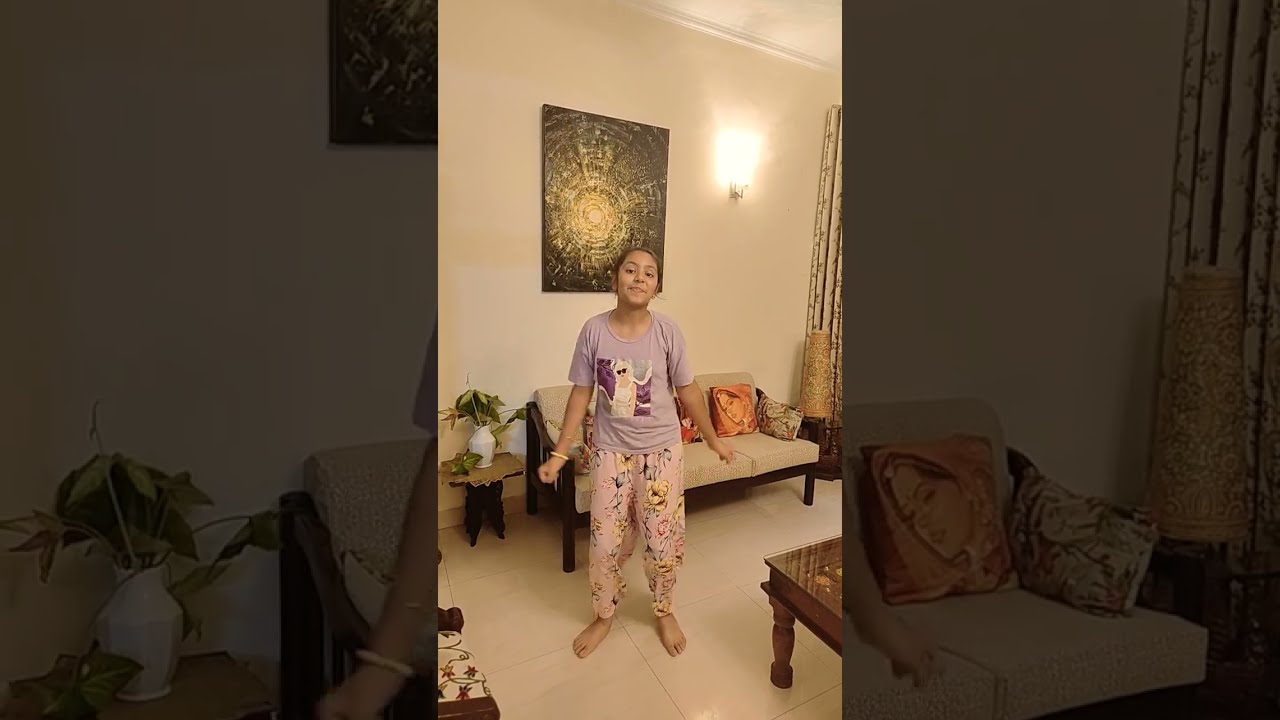The image is a vertical cell phone picture centered within a landscape that is divided into thirds, surrounded on both sides by a zoomed-in and faded version of the main image. The central photo features a teenager, likely under 20, with medium skin tone and dark brown hair pulled back, standing in a room in her pajamas. She is wearing a purple shirt with an indistinct white graphic and pink pajama pants adorned with yellow figures. The floor she stands on is a hard, beige colored surface. Behind her is a dark tan couch with purple pillows resting against a beige wall. Above the couch hangs a round, gold, abstract painting that resembles a sun. To the left side of the couch is an end table with a plant. There's a light fixture on the right side of the wall that is switched on, casting a glare. The girl appears to be smiling with her mouth closed and her hands slightly out to her sides. Her feet are bare. In the foreground to the left of the image, there's a coffee table, and other pieces of furniture can be partially seen.